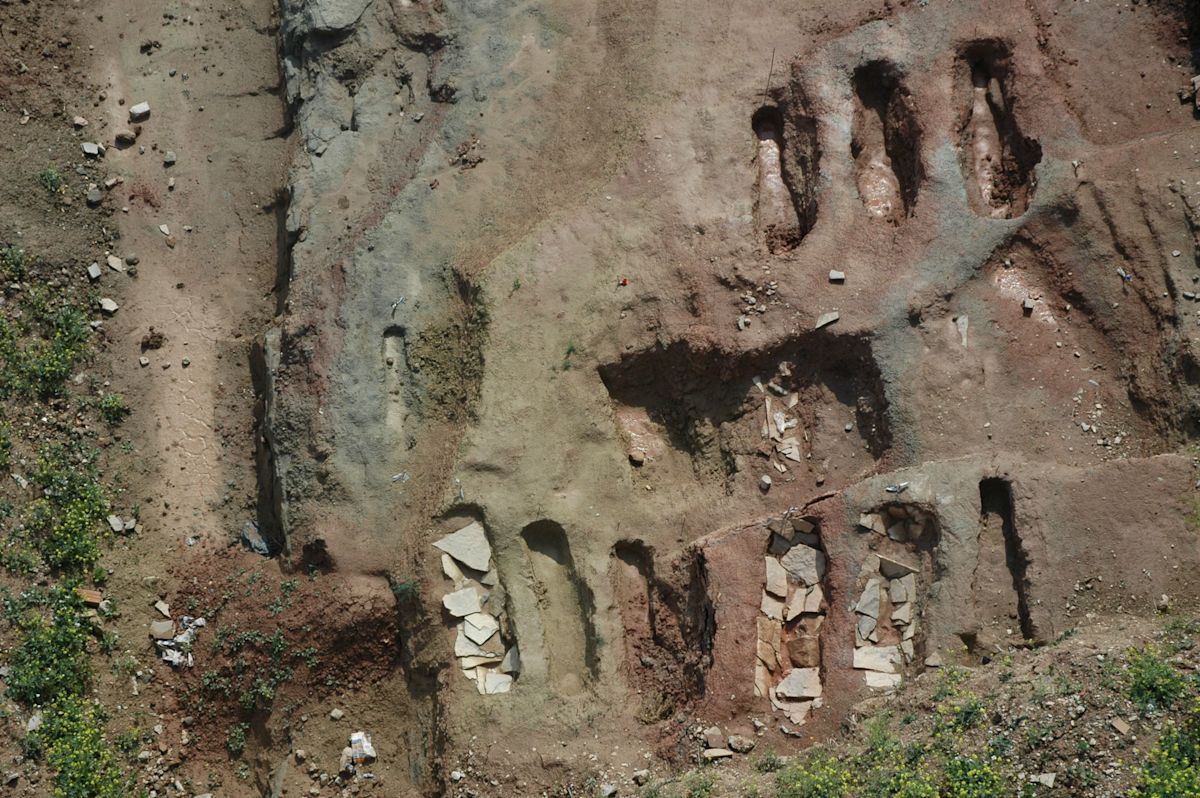The photograph, taken outdoors during the daytime, captures an aerial view of an excavation or archaeological site with a rectangular shape approximately six inches wide and three to four inches high. The focal point of the image is a weathered rock formation with seven distinct vertical rectangular cutouts. 

At the top of the formation, there are three additional vertical rectangles. Below them, a large horizontal rectangular indent spans across. The central portion seems filled with large white rock pieces, particularly noticeable in the first, fifth, and sixth cutouts, while the third and fourth are visibly connected and contain darker soil.

Surrounding this formation, the landscape comprises layers of varied soil colors - reddish, light brown, and bluish dirt. Ledges with green foliage and light yellow flowers are present on the left edge and the lower right corner of the photo. The terrain, dotted with stone or pottery fragments, further emphasizes the meticulously dug-out depressions resembling graves.

To the right of the scene, the ground is characterized by brown patches and debris, hinting at a possible road. The left and upper portions of the photograph include elevated areas that cast shadows, adding depth to the image and highlighting the intricacies of the excavation site.